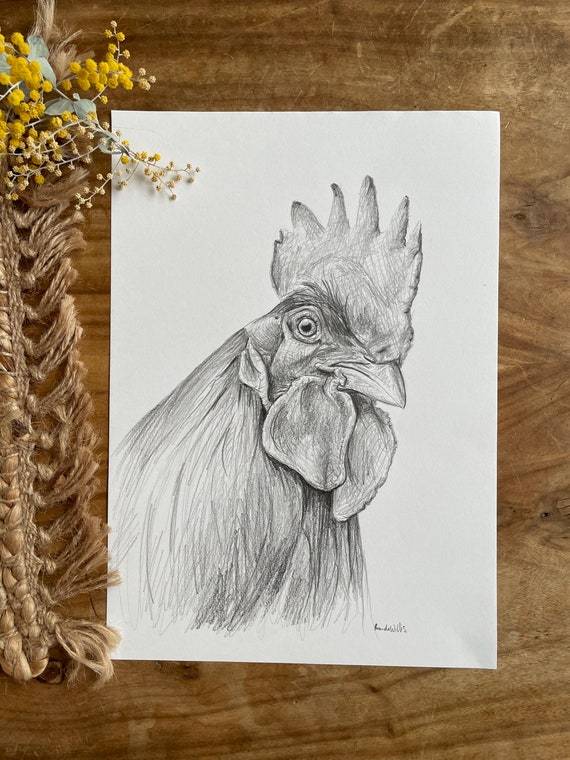This photograph captures a detailed, hyper-realistic pencil sketch of a rooster, positioned atop a wooden tabletop with visible wood grain. The rooster's head and neck are meticulously rendered, showcasing its red comb and wattle, with dark feathers cascading down. The rooster's piercing gaze is directed forward, and a small, unreadable signature of the artist appears toward the bottom right of the sketch. The drawing is on a pure white sheet of paper. To the left of the paper lies a decorative macrame item made from either rope or braided yarn, colored brown, and a small plant with yellow flowers and light green leaves, adding a natural touch to the composition.